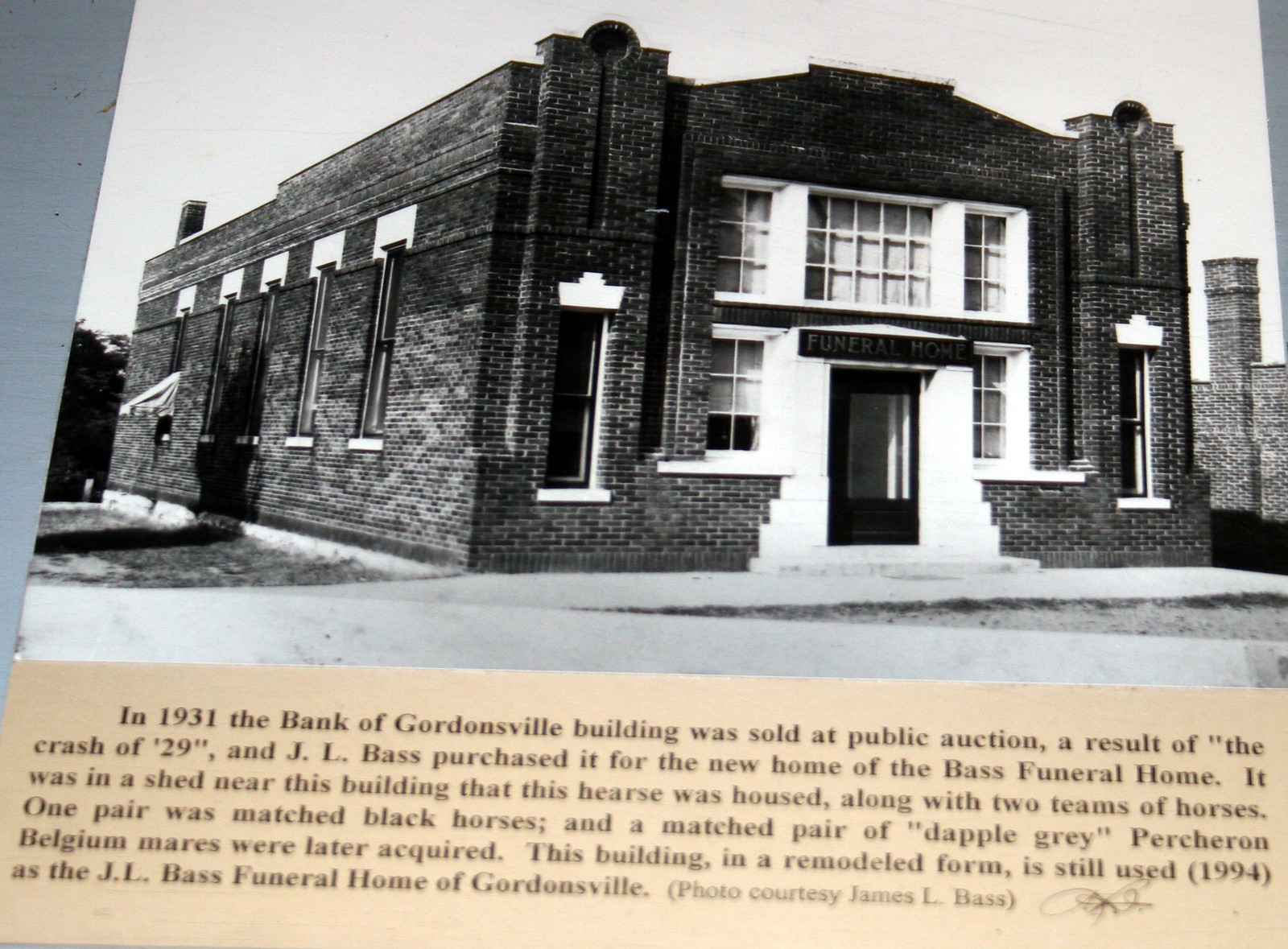This black and white photograph depicts a large brick building that was once the Bank of Gordonsville, converted into a funeral home. The building is characterized by a central black door with a window, flanked by white wooden columns that extend down to the sidewalk. A black sign above the door clearly reads "Funeral Home." The façade of the first floor features white-shuttered windows on either side of the door, which are vertically rectangular, approximately four to five feet high and one to two feet wide. The second story also has windows directly above these, maintaining a symmetrical appearance. 

The left side of the image shows part of the building's side, with four additional windows, one of which has an awning. In the background, there is another brick structure resembling a turret. Underneath the picture, on a light beige box with black text, the caption reads: “In 1931, the Bank of Gordonsville building was sold at public auction as a result of the Crash of '29. J.L. Bass purchased it for the new home of the Bass Funeral Home. This building has been remodeled and was still in use as the J.L. Bass Funeral Home of Gordonsville as of 1994. This hearse was housed in a nearby shed, originally kept with two teams of horses: one pair matched black and another pair matched gray. Photo courtesy James L. Bass.” The detail and history provided in the caption enrich the visual narrative of this well-preserved historical structure.